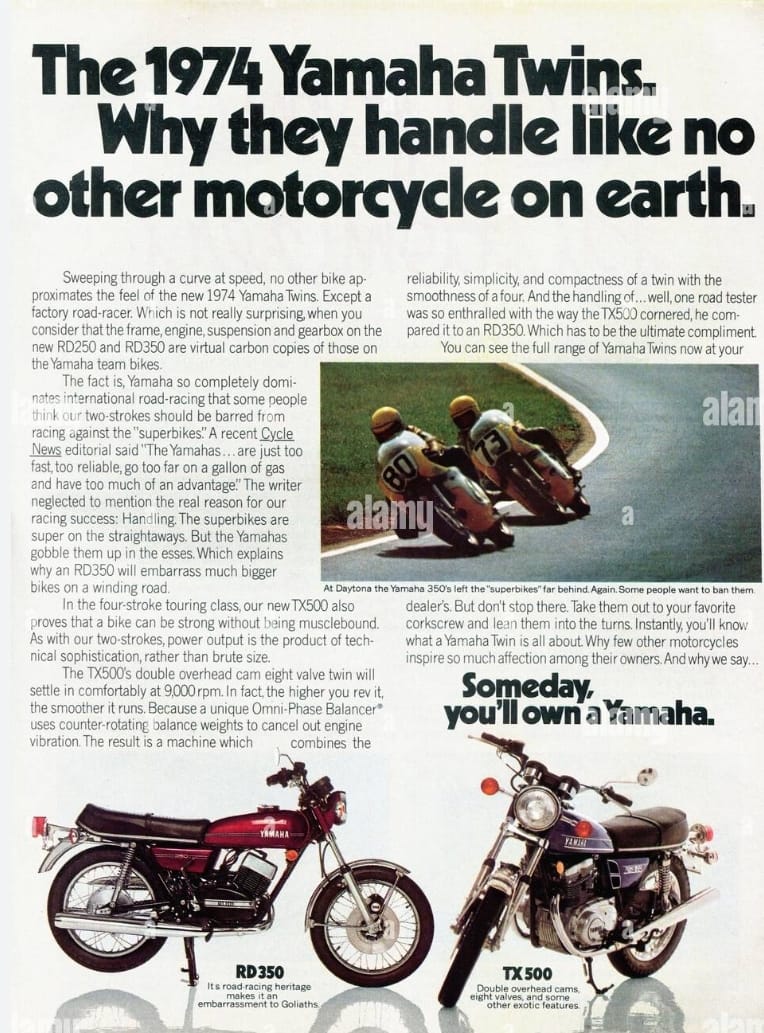The image shows a detailed poster or magazine page dedicated to the 1974 Yamaha Twins, specifically models RD250 and RD350. The heading at the top, "The 1974 Yamaha Twins: Why they handle like no other motorcycle on earth," is prominently displayed in large black letters. Below this, the text elaborates on the exceptional performance and design of these motorcycles, which are said to replicate factory road racers closely.

The layout features four paragraphs on the left side and another paragraph at the top right. Beneath the top-right paragraph, there is a vivid image of two riders, showcasing the motorcycles in action on a track. The bottom of the page includes pictures of two motorcycles: the red RD350 on the left, facing right, with a black seat and handlebars, and the blue TX500 on the right, facing left with the front tire angled toward the viewer, detailed with a blue chassis, blue highlights, and a significant amount of chrome. Each motorcycle image is accompanied by black numbering and some text beneath, though these details are less legible. Additionally, the bottom right corner of the page features the phrase "Someday You'll Own a Yamaha" in bold black text. 

The overall tone and style suggest an informative and promotional article highlighting the advanced features and superior handling of the 1974 Yamaha Twins models.